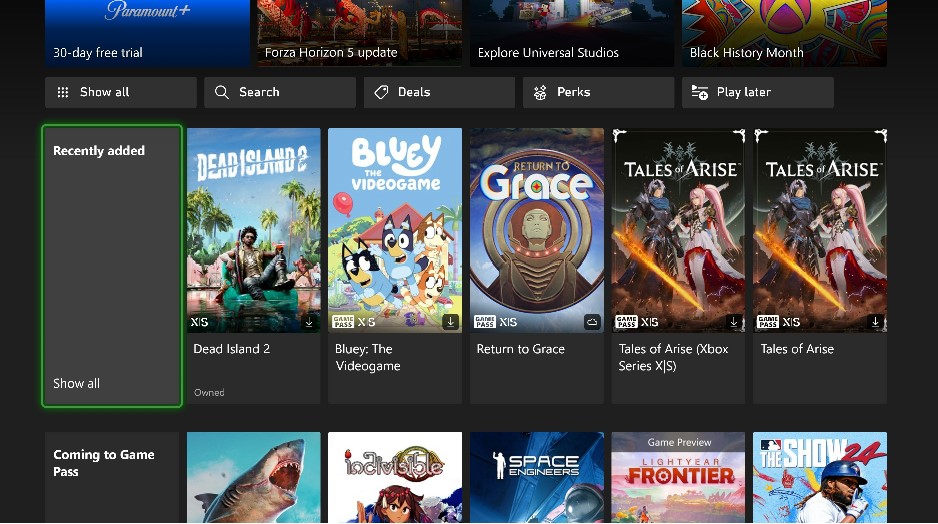The screenshot showcases a curated selection of video games presented in vertically oriented rectangles, each featuring a thumbnail of the game’s artwork along with its title. The highlighted titles include "Bluey: The Video Game," "Return to Grace," "Dead Island 2," and "Tales of Arise" for Xbox Series. At the top of the page, a grey box with white text reads "Recently Added Show All," indicating that these games have recently been added to the collection.

Beneath this, a secondary row displays video games that are soon to be available on Game Pass, consisting of five different titles. Among these forthcoming releases are "Space Engineers" and "Lightyear Frontier," the latter of which includes a game preview option. Additionally visible are a title featuring a shark on the cover and "MLB The Show 24."